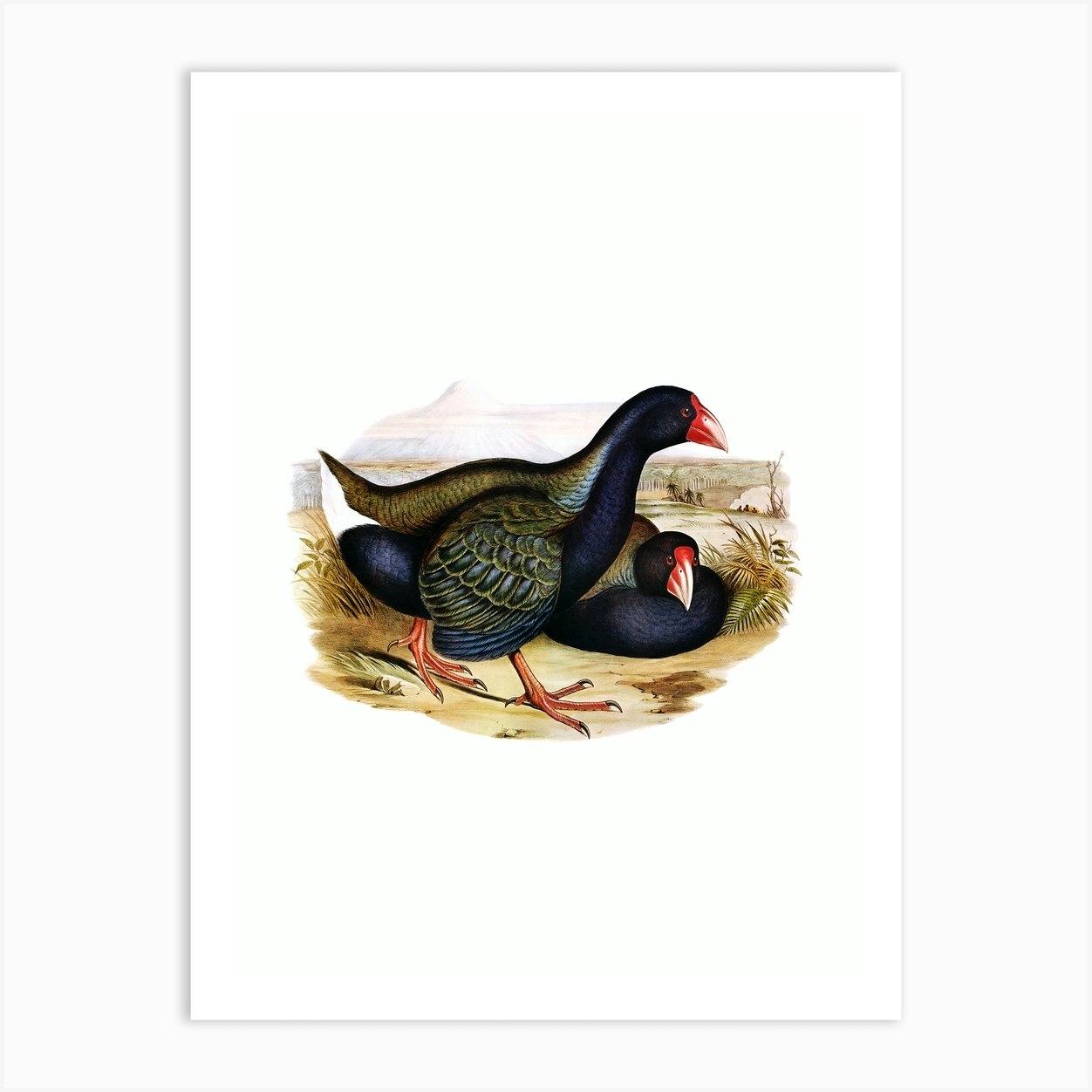This is a vertical, rectangular image set against an off-white background, featuring a smaller white rectangle in the center that contains a detailed drawing or painting. The artwork depicts two birds, possibly ducks, characterized by their distinctive red and pink beaks with white tips, black bodies, and golden-black wings. Their talons are orange. One bird stands and walks towards the right, while the other lies on the ground, also facing right, appearing relaxed. The ground is depicted in brownish-gray tones, evoking a desert-like, possibly weedy landscape. The sky above the birds is a light blue with hints of pink, adding to the serene atmosphere of the scene.